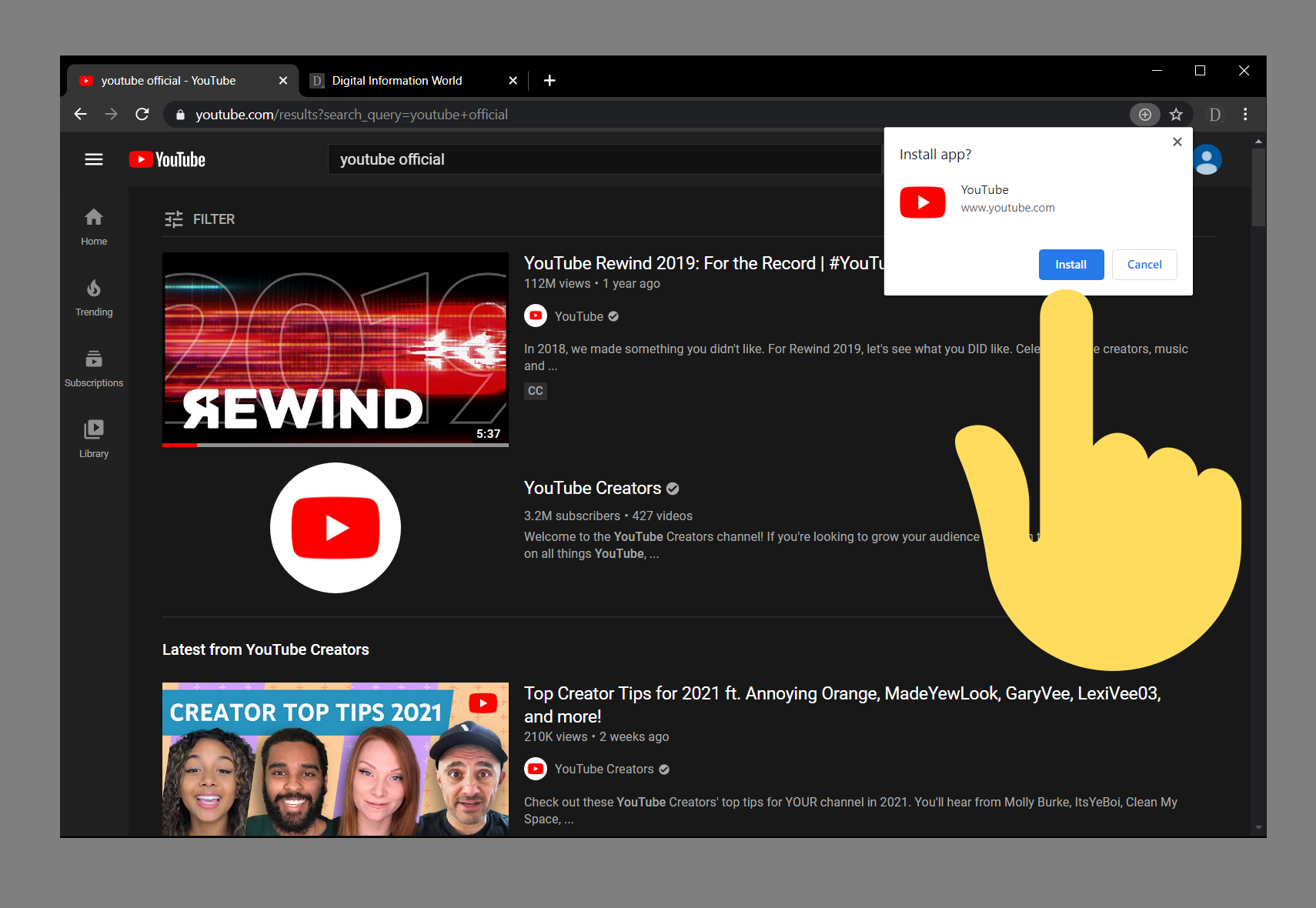In this screenshot taken from the YouTube website in dark mode, a prominent yellow Android-style hand emoji is positioned on the right side of the image. The hand is making a gesture with the thumb and pointer finger extended, directing attention to a pop-up message. The pop-up, which is urging the user to install the YouTube app, includes an option to "Install" or "Cancel," with the finger specifically pointing towards the "Install" button.

The screenshot also shows the user has two browser tabs open: one labeled "YouTube official" and the other "Digital Information World." The background, typical of YouTube's dark mode, is predominantly black and grey.

Visible within the screenshot are recommendations for YouTube videos, including "YouTube Rewind 2019" and "Top Creator Tips for 2021" featuring creators like Annoying Orange, Madey Look, Gary Vee, and Lexi VO3. Both videos are attributed to YouTube Creators, indicating they were produced by YouTube's own team to highlight platform content and creator tips.